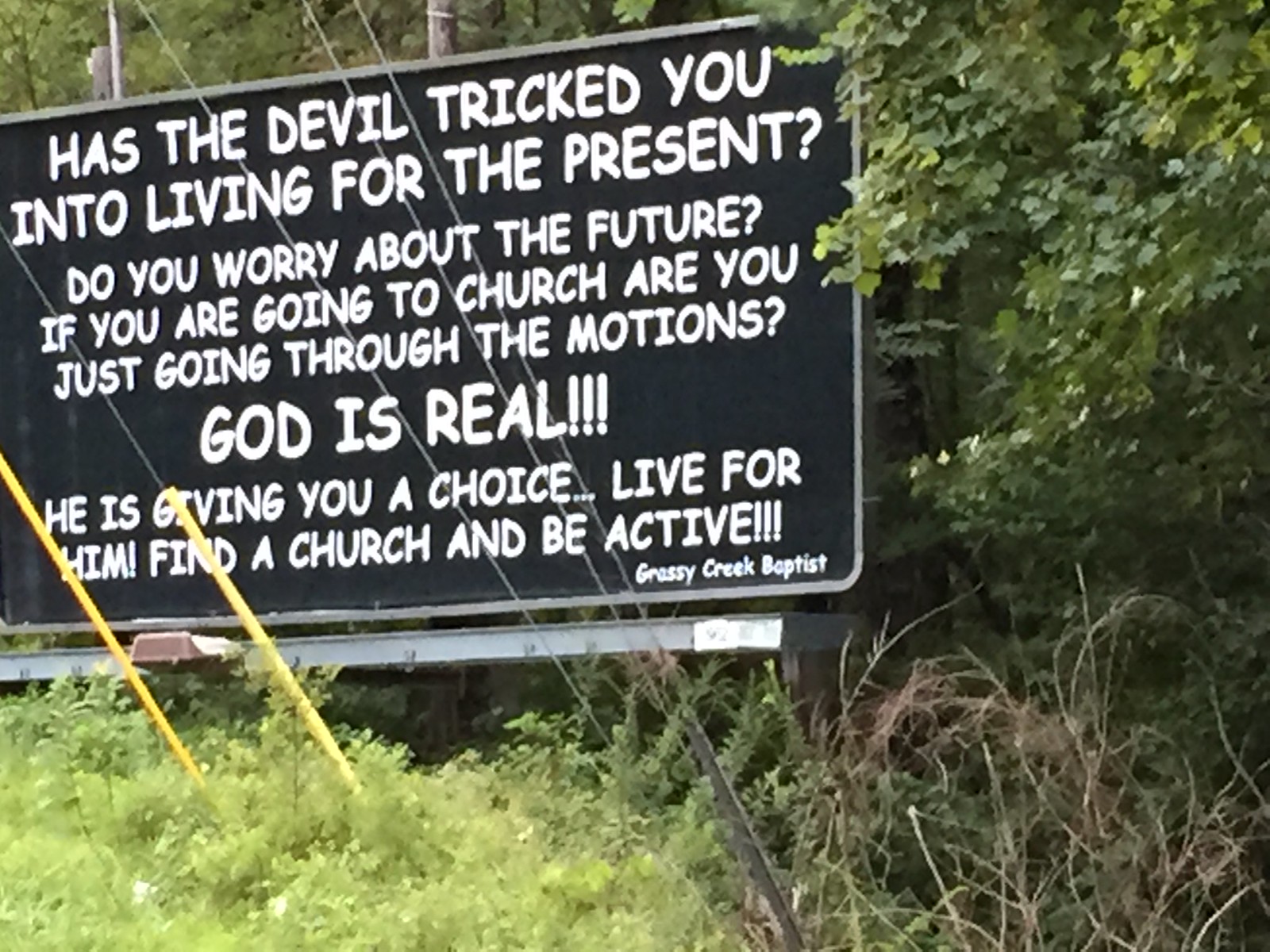This photograph captures a solitary billboard erected amidst a dense, lush forest of vibrant green trees, interspersed with bushes and grasses. The billboard, matte black in color, starkly contrasts with its verdant surroundings. Emblazoned across the board in bold white text are thought-provoking questions and statements: "Has the devil tricked you into living for the present? Do you worry about the future? If you are going to church, are you just going through the motions? God is real. He is giving you a choice. Live for Him. Find a church and be active." At the bottom, the sign is attributed to Grassy Creek Baptist. The vivid greenery framing the billboard accentuates its message, creating a striking depiction of spiritual outreach amidst nature's embrace.